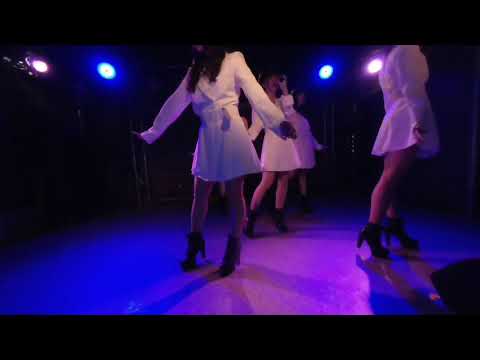In a dimly lit stage scene bathed in blue and purple hues, four women are captured mid-dance routine, their elegant movement accentuated by the dramatic lighting. The stage lights cast directional beams, creating shadows that dance along with the performers. Each dancer is dressed uniformly in white, raincoat-style long-sleeved dresses that are hemmed above the knees, cinched at the waist with a belt. Complementing their attire are tall, black, chunky high-heeled boots, adding a stark contrast to their outfits. Their poses vary: the woman in the front on the left has her head cut off by the edge of the image, while the one next to her reveals just a part of her face and long dark hair draping below her shoulders. The two women in the back are partially obscured—one by her own hand and the other swallowed by the shadows, enhancing the photo's mysterious and moody atmosphere.